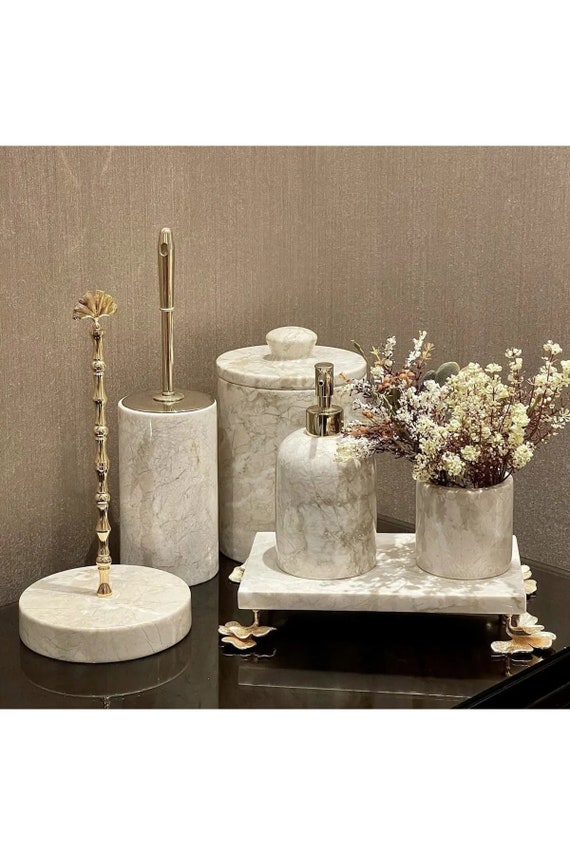This photograph captures an elegantly arranged set of bathroom decorations on a sleek, black reflective table surface, set against a textured brown wallpaper with vertical stripes. The tableau is composed of five ivory marble decor pieces, each detailed with luxurious materials such as gold and silver. 

On the left, a circular marble base supports a golden tower topped with a decorative golden fan. Beside it and slightly to the right stands a taller, slender marble cylinder. This piece features a silver top and a smooth silver dowel protruding from it, complete with a small hole at its very tip.

Continuing rightward, there’s another cylindrical marble container, taller and broader than the previous, capped with a marble top and a small button handle. At the far right of the table, a raised marble slab with golden leaf feet holds two items: a marble soap dispenser with a rounded top and silver pump on the left, and a marble vase filled with pale yellow flowers with red stems on the right. All these marble pieces share an identical creamy design, exuding opulence and refined taste.